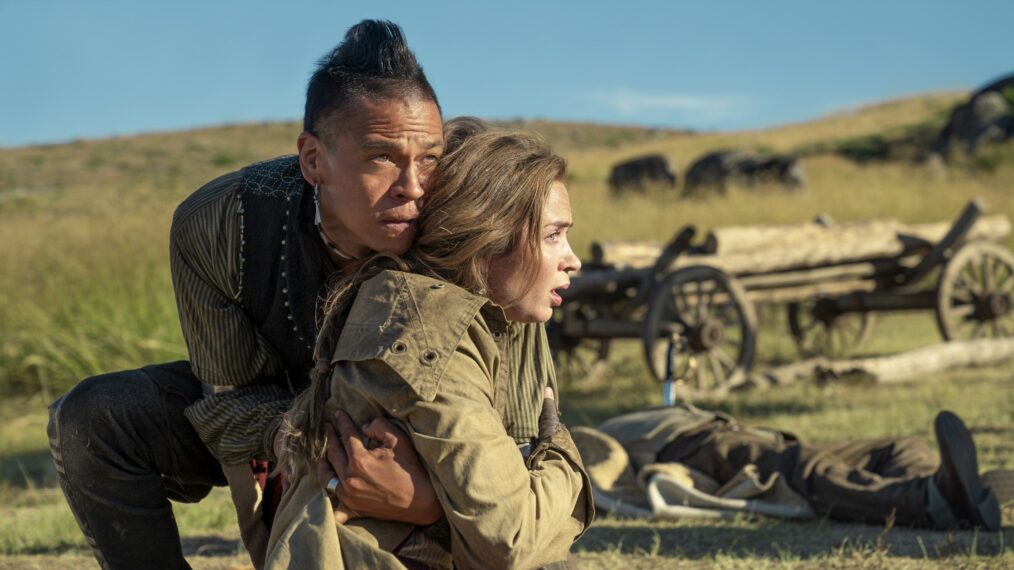The image captures a tense moment in an open prairie with tall grasses in the background and possibly animals grazing in the distance. At the center of the scene, an indigenous man in a striped shirt, vest with beadwork, and blue jeans, is holding a white woman with long brown hair who is wearing an olive-colored jacket. They are both in a crouched position, with the man down on one knee, and both are looking off to the right with expressions of fear and concern. The woman has her hands wrapped around herself, clearly in shock. Behind them lies a person dressed in a gray shirt and brown pants, seemingly lifeless or unconscious, with shoes still on and a blanket underneath. Off to the side, an old wagon loaded with long logs suggests that they were building a structure. The overall scene appears to be a dramatic still from a movie.